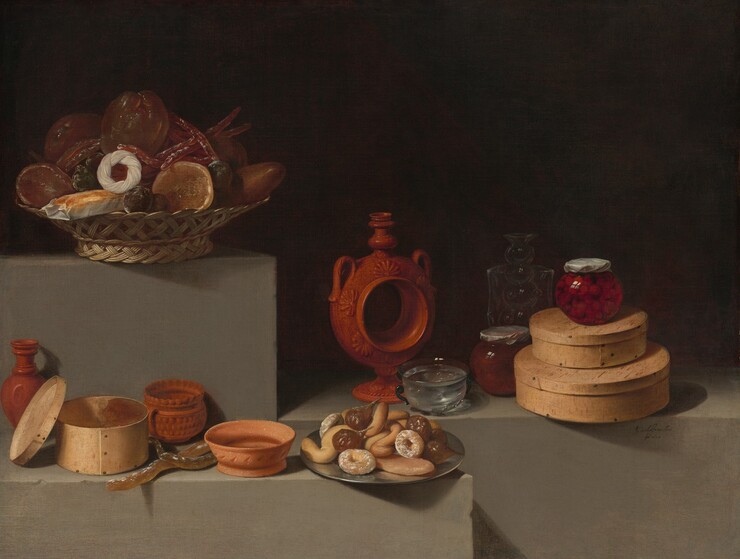In this dark-toned image, the primary focus is on a variety of pottery, baskets, and food items arranged intricately on different gray concrete blocks, lending an artistic and almost antique feel to the scene. In the upper left-hand corner, a wicker basket holds an assortment of circular objects, possibly dried oranges and red items, elevated on a gray box. 

In the foreground, there's a striking red vase with a large circular middle that you can see through. Adjacent to it, a brown circular box has its lid off and propped on its side. The lower part of the image contains two brown bowls and other baskets. A silver plate filled with various baked goods such as doughnuts, pastries, and potentially long bread is prominently placed in the center. These baked items are in shades ranging from light tan to dark brown, some dusted with powder.

To the right in the background, two hat boxes serve as a platform for more containers, including a clear glass jar that appears to contain some kind of jelly, and a red jar of what looks like jam. The jars and containers, which appear to be a mix of clear glass and reddish, orangish pottery, are reminiscent of ancient Roman or Greek artifacts. 

Overall, the composition, with its various containers and food items spread across gray stones, evokes a sense of timelessness, blending elements of history, art, and culinary delight.